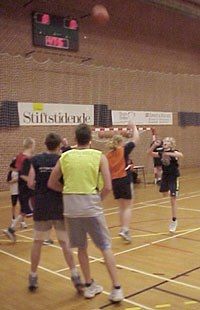The image depicts a small, unclear snapshot of what appears to be an indoor athletic game, likely netball, taking place on a polished brown court. The scene is set in a gymnasium, identifiable by the scoreboards mounted on the walls and various advertisement billboards surrounding the perimeter. The floor is marked with lines indicating the boundaries and zones of the court. At least six individuals are gathered closely together in the frame, all sporting a variety of colored clothing including red, yellow, orange, and black, which makes it difficult to discern any specific teams or organized play. There is no visible net or ball, suggesting that this may be a practice session or some form of exercise rather than an official game. Overall, the setting seems lively yet somewhat unstructured, contributing to the impression of an exercise session rather than a competitive match.